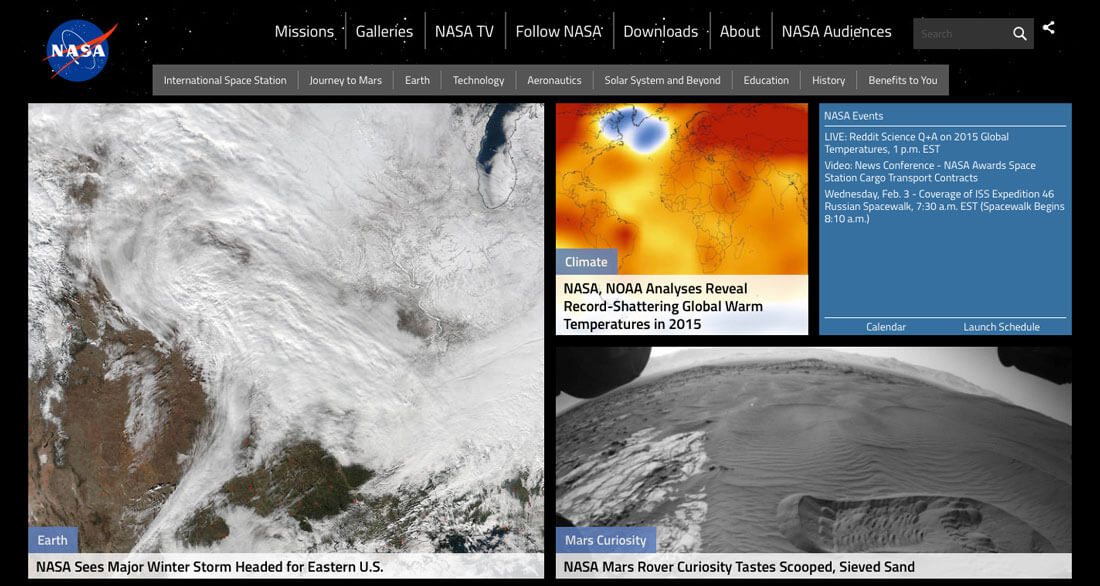The top left corner features the distinctive NASA logo, which consists of a circular blue symbol with a red swoosh. Adjacent to it on the navigation bar, you'll see categories such as "Missions," "Galleries," and "NASA TV." On the far left, there is also "About NASA," a search bar, and a search button.

Prominently displayed on the page is a weather map depicting a significant winter storm. The headline reads, "Major Winter Storm Headed for Western U.S.," under the section titled "Earth in Time." Alongside this, another map labeled "Climate" presents a thermal analysis. A noteworthy article highlights, "NASA Analysis Reveals Record-Shattering Global Warming Temperatures in 2015," signifying the gravity of climate change.

The page further advertises upcoming NASA events. For instance, a live Reddit Science Q&A on 2015 global temperatures is scheduled for 1 p.m. Eastern Time. There's also mention of a daily news conference, "NASA Awards," details about the Space Station's cargo transport scheduled for Wednesday, February 3rd, with subsequent cargo drives on February 4th and 6th. The calendar and the launch schedule are also prominently highlighted.

Near the bottom, the page features a breathtaking image of the Martian surface under the heading "Mars Curiosity." The desert-like landscape is accompanied by the caption, "NASA's Mars Rover Curiosity Tastes Scooped Sea Sand." The overall background of the page is rendered in a deep black, enhancing the contrast and visual appeal of the featured images and text.